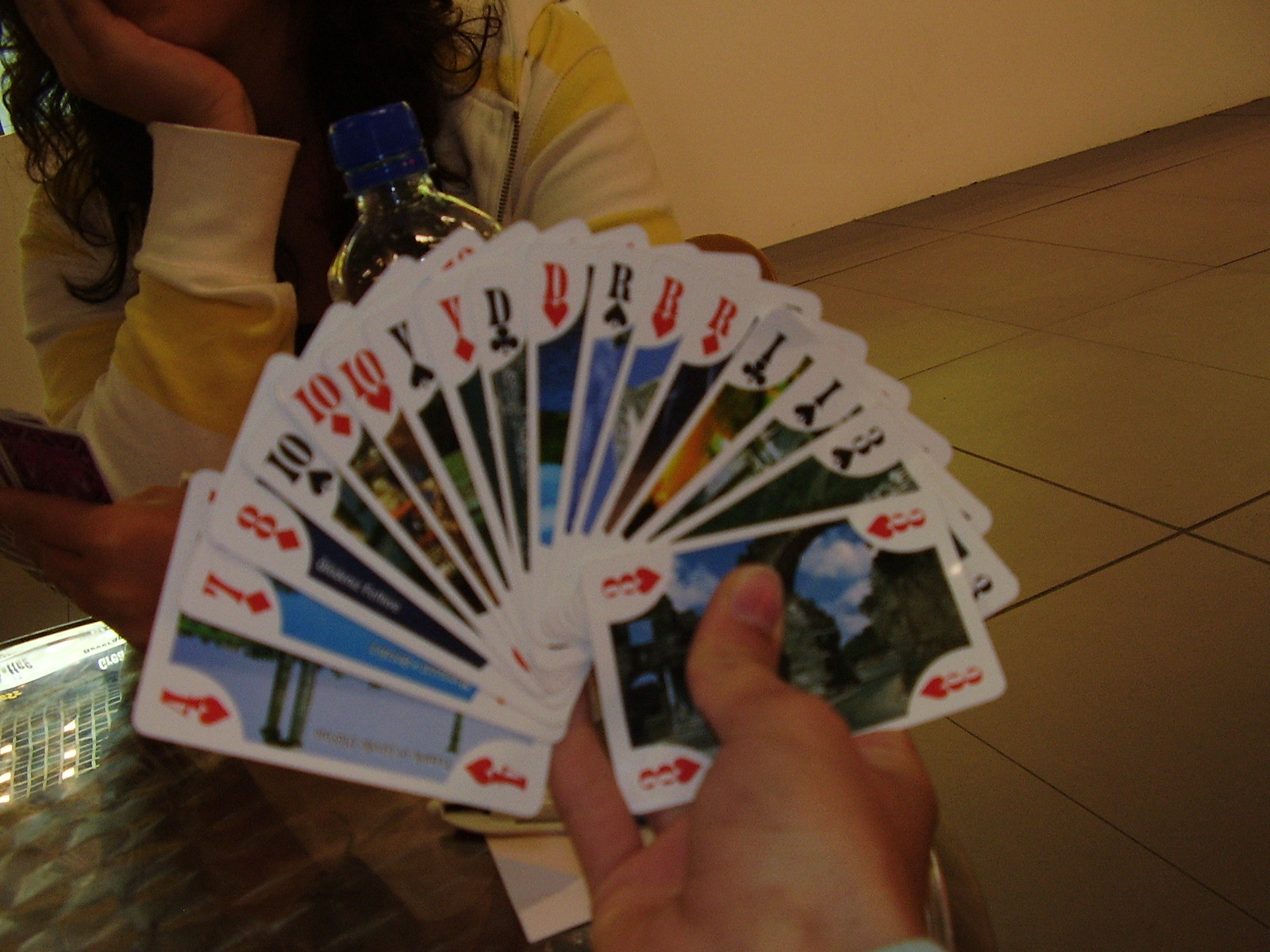The image depicts a couple engaged in a card game, viewed from the perspective of one player holding a hand of cards. The hand, which could belong to either a man or a woman, contains roughly 15 cards from a deck that includes traditional suits like hearts, clubs, spades, and diamonds. However, the deck also features unusual cards labeled with letters such as V, D, R, and I, in addition to commonly recognized cards like the seven of diamonds, eight of diamonds, and four of hearts.

Across the table, the person's opponent, presumed to be a woman based on her visible hair, build, and hand appearance, also holds a set of cards. She appears to be focused intently on her hand. The game is being played on a tiled table, with a water bottle placed centrally between the two players, suggesting a casual and relaxed setting for their activity.